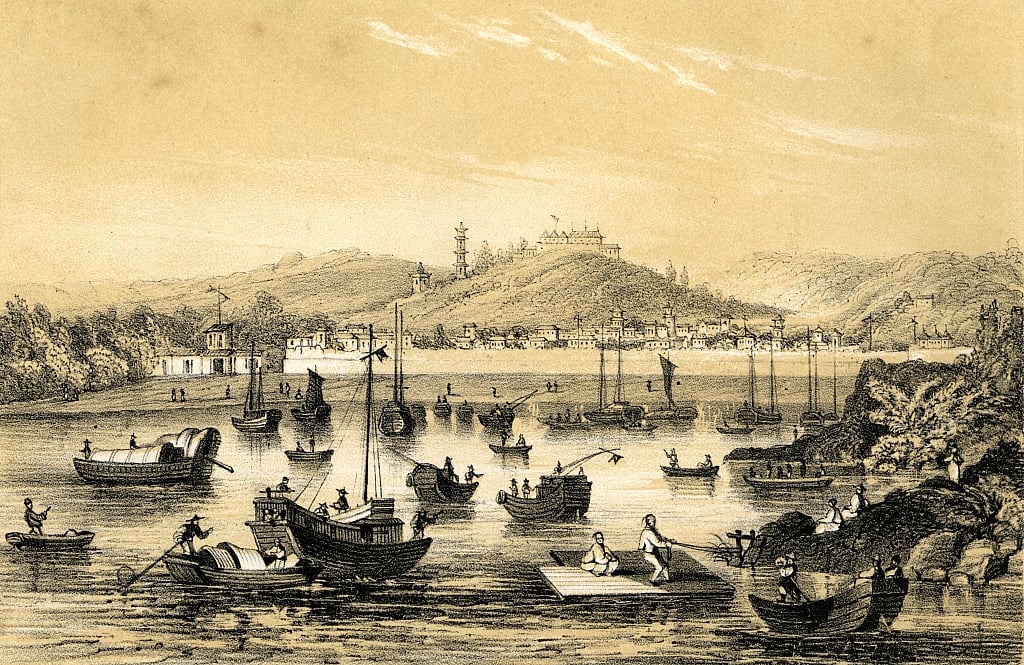This image is an older sepia-toned painting that appears to depict a bustling scene from an ancient settlement, possibly in China. The composition features a grand temple or fort with layered roofs sitting atop a prominent hill, dominating the background. Further behind, rolling hills extend into the distance. In the valley below, a small town with numerous homes is spread out, offering a glimpse into the local life of the period.

The foreground is dominated by a large body of water, teeming with a variety of watercraft. There are numerous boats of different sizes, including sailboats, rowboats, kayaks, canoes, and even simple rafts with people aboard. The water is bustling with activity, suggestive of a vibrant community or marketplace, and several figures appear to be fishermen or townspeople loading boats. A small rocky island is situated to the right, adding to the intricate detail of the scene. Overall, the artwork masterfully captures a moment in time, highlighting the intersection of natural beauty and human endeavor.